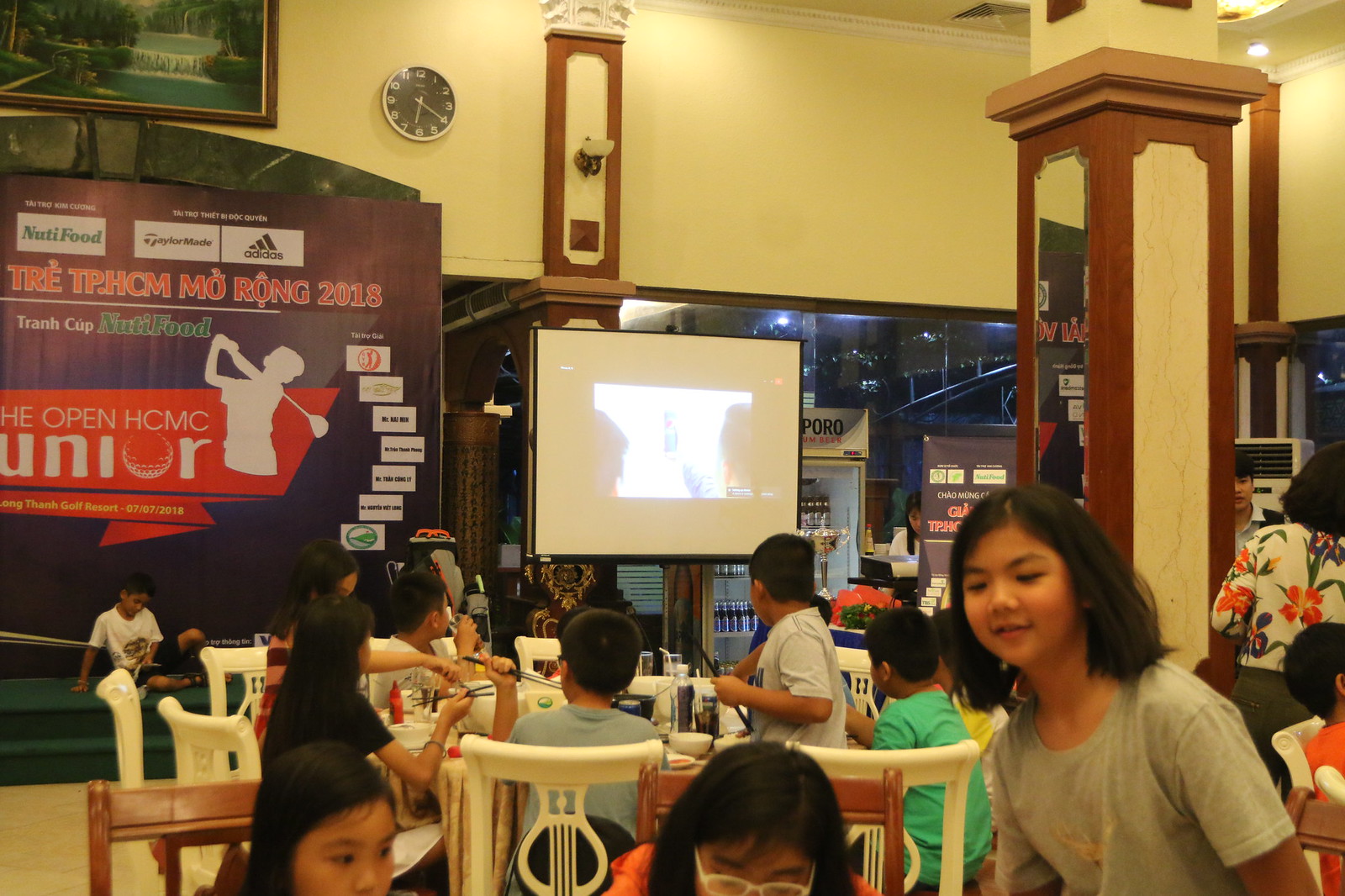The image depicts an indoor setting where a social event is taking place, possibly in a restaurant, convention center, or assembly hall. The room is brightly lit with indoor lighting, featuring tan walls, wooden trim, and white chairs. Multiple tables are arranged around the space with a number of people, primarily young individuals, seated and engaged with the surroundings. Predominantly, attendees have dark hair and are wearing white and black shirts, with many focused on a screen set up in the background, possibly displaying a movie or video.

Central to the scene are a few individuals close to the camera, including an older woman and a young child on the left, as well as another woman in the middle and right. This central grouping stands out against the backdrop of the event. Notably, a small green stage is visible to the left, featuring a boy seated on it and a sign bearing some recognizable logos like Nutri-Food and Adidas, though much of the text is in a non-English language.

An advertisement for a junior golf club is prominent in the upper right section of the room, characterized by a red block with white writing and the silhouette of a person swinging a golf club. Additional details include a tall column to the right with a mirrored section, and a black analog clock on the wall reading 6:20. The space also features tall windows through which darkness outside can be seen, enhancing the indoor ambiance.